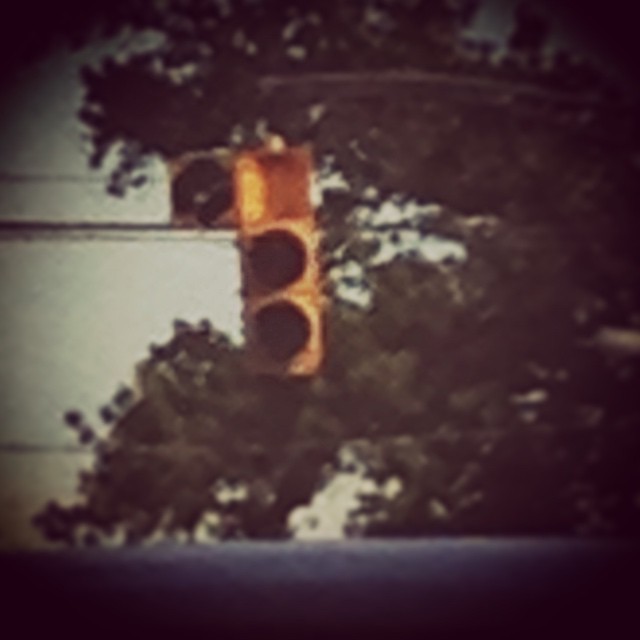This photograph depicts an old and faded stoplight, appearing out-of-focus and drawn from a bygone era with colors reminiscent of the 1960s. The traffic signal is clearly broken; its top light, which would typically display red, is dislodged and flipped to the left, revealing an empty and open housing. The remaining lights are intact but unlit. The stoplight is suspended from a metal rod with visible power lines running through the frame. In the background, one can discern the outlines of tree branches with leaves and a patch of sky, adding to the vintage, somewhat somber atmosphere of the image.